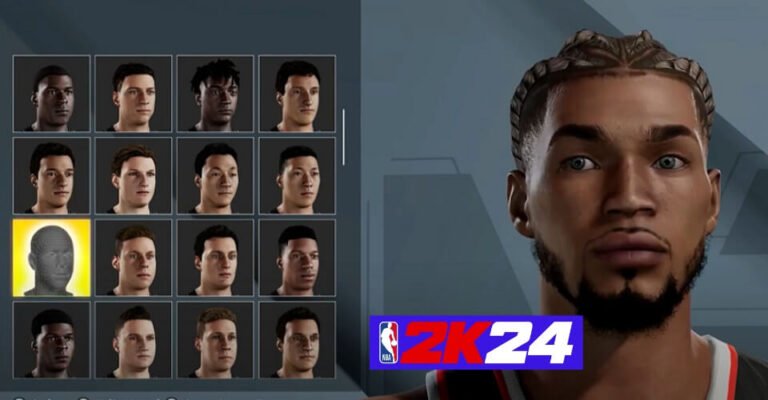This image is a detailed screenshot from the video game NBA 2K24, specifically from the player customization screen. On the left side of the screen, there is a 4x4 grid displaying 15 different customizable player faces, representing various races and skin tones. Each option features players with short hair, except for the highlighted selection. The selected option is marked by a silhouette of a head against a yellow background in the grid. On the right side of the screen, a close-up view shows an African-American man with braided hair, a beard, and medium-toned skin, dressed in a basketball jersey. The game’s logo is prominently displayed with a blue bar, featuring bold red "2K" and white "24" text, accompanied by the NBA logo on the left-hand side.